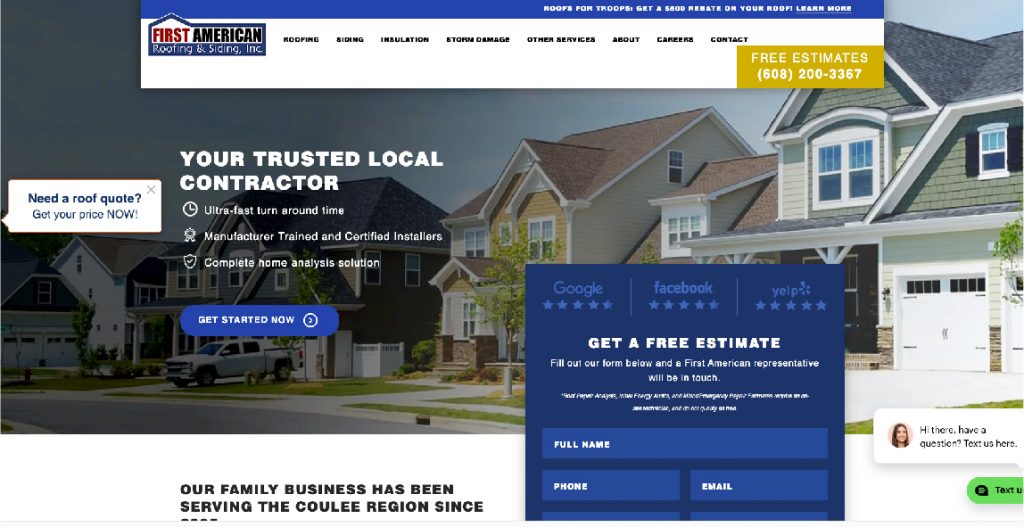**Caption:**

A screenshot from a home builder or contractor's website showcasing a residential neighborhood in the U.S. or Canada with fairly new homes characterized by gray asphalt or shingle roofs and tan to black exterior colors. On the left side, a large white truck is parked in a driveway. The website features a blue banner at the top with white text that is not fully legible. Below, there's another banner with a white background on the left, displaying a blue house icon and the words "American First." 

Prominent in the center is a bold yellow text offering a "free estimate" accompanied by a contact phone number. A white box within a housing image on the left reads, "Need a roof quilt? Get your quilt now," followed by "You're a trusted local contractor" in white text. Additional information includes promises of an "ultra-fast turnaround," and "trained and certified" services. 

A noticeable purple pop-up in the center prompts users to get their free quilt by entering their first name, last name, and email address. To the left of this pop-up, there is a message in black text stating, "Our family business has been serving the Cooley region since..." although the rest of the sentence is cut off.